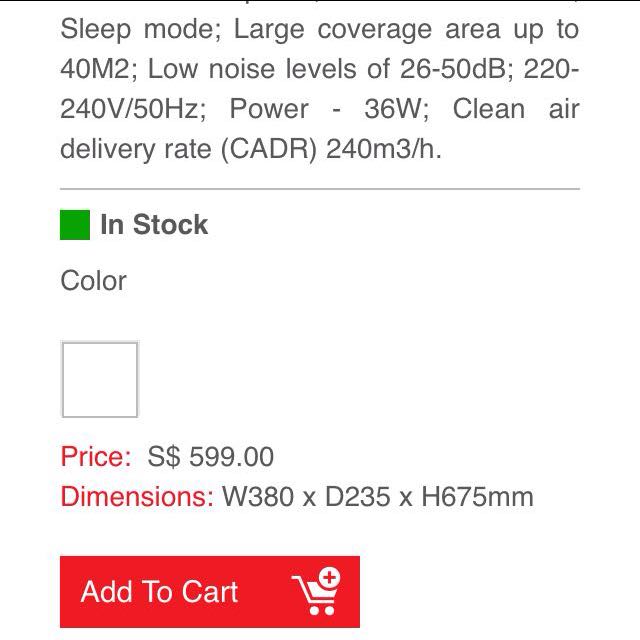Screenshot of a Portion of a Website with Product Information

The background of the image is white. At the top, there is a thin black line running horizontally across the entire screenshot. Just below this line, the following product specifications are listed in bold black font:

- Sleep mode;
- Large coverage area up to 40m²;
- Low noise levels of 26-50dB;
- 220-240V / 50Hz;
- Power: 36W;
- Clean Air Delivery Rate (CADR): 240m³/h.

Beneath these specifications is another horizontal black line. Below this line, there is a red square positioned to the left. To the right of the red square, the words "In Stock" are displayed prominently in bold black font. 

Underneath this, the word "Color" appears in black font, followed by an empty white square, indicating a potential color selection option. Below the empty square, the price is listed in red font as "S$599.00."

Finally, at the bottom, the dimensions of the product are stated in black font as "Dimensions: W380 x D235 x H675mm".